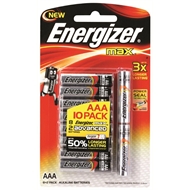This is a detailed caption for the image of the pack of Energizer batteries:

"A pack of Energizer AAA batteries prominently displayed in its retail packaging. The top left corner features the word 'NEW' in bold yellow uppercase letters. Below this, a small punch hole allows the package to be hung on store shelves. The brand name 'Energizer' is boldly printed in white with a capital 'E', set against a black background patch that stands out on the packaging. The design flows with deep orange and light streaks, transitioning to yellow near the bottom and culminating in white at the far right corner.

Under the Energizer logo, the word 'MAX' appears in yellow, and just to the right and slightly below, it reads '3x Power'. An animated battery character is seen running towards the batteries, giving a dynamic look to the packaging. A yellow sticker at the bottom reads 'AAA 10 Pack' in red letters. Beneath this sticker, the word 'ADVANCED' can be faintly seen in white. Near the bottom of the label, the number '50%' is partially visible in white text on a black background, though the rest of the text is unclear due to blurriness. In the bottom left corner, 'AAA' is printed again in black.

The pack contains a total of 10 AAA batteries, stacked in two columns: eight batteries are arranged vertically one above the other on the left, while the remaining two are positioned similarly to the right of the main column, also stacked vertically."